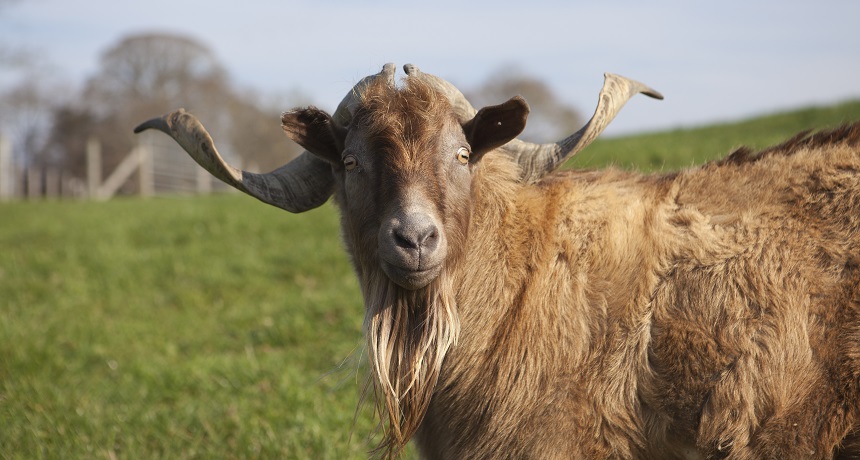In the foreground, a majestic longhorn sheep gazes directly at the camera. The sheep, positioned slightly to the right and extending towards the center of the image, boasts a light brown coat and impressive, intricately twisted horns. Its face, adorned with light brown eyes and black pupils, features erect, rounded ears and a tan-colored mouth, nose, and chin area. The chin is embellished with a beard of long, light brown hairs.

Behind the sheep stretches a lush grass field, leading to a wire fence and gate on the left side of the background. Beyond the fence, a cluster of trees marks the horizon under a gray, overcast sky. This detailed composition captures the serene yet striking presence of the longhorn sheep amidst its natural habitat.